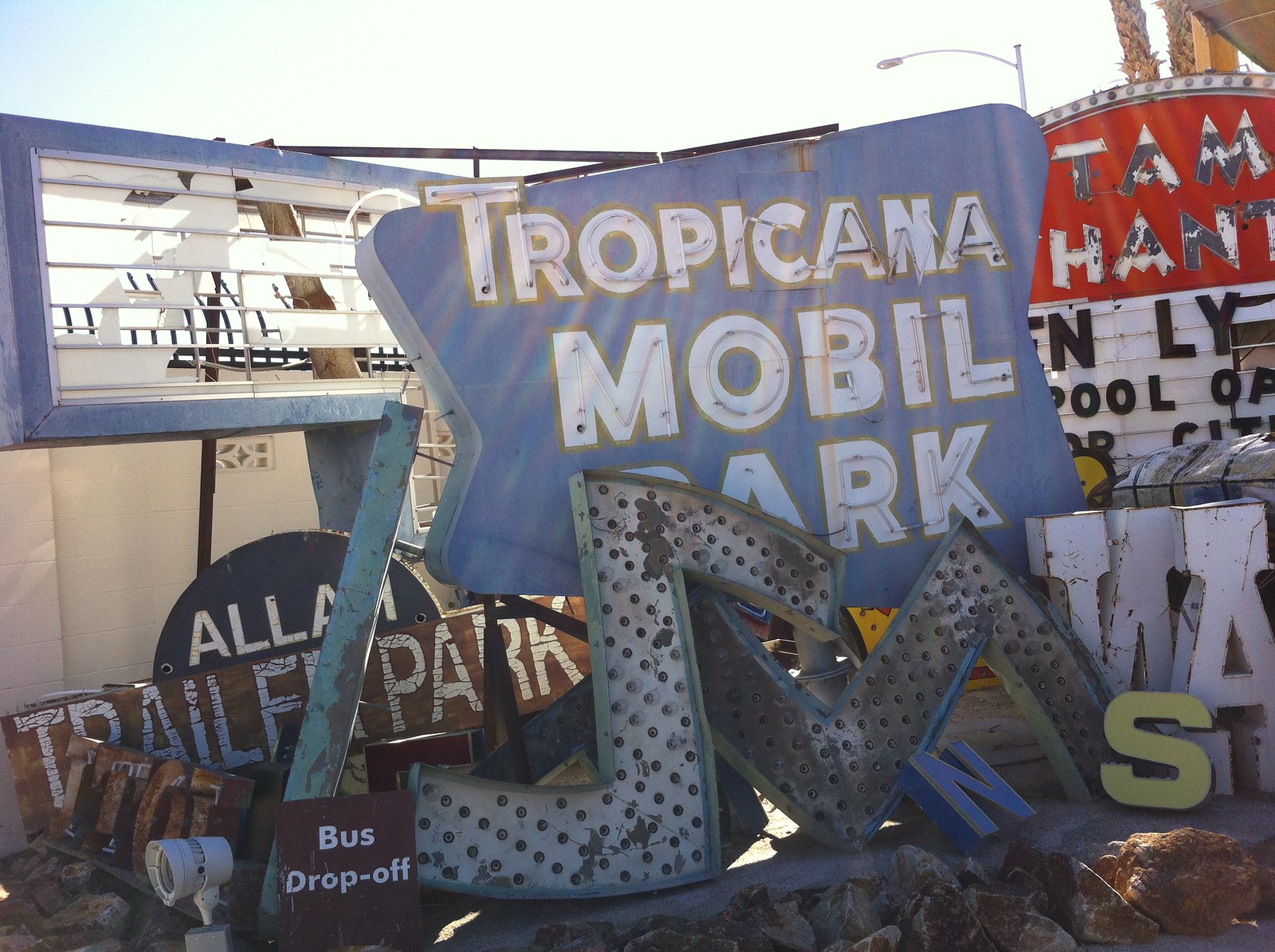The image shows a junkyard of old, discarded amusement park and plaza signs, many of which are damaged and dirty. Central to the image is a large, weathered blue sign with three lines of white text reading "Tropicana," "Mobile," and "Park," hinting at its past vibrancy. Nearby, a brown "BUS DROP OFF" sign lies in the bottom left corner, and a half-circular sign that says "ALAM" or "ALUM" appears to the upper left. In the upper right, an arched red sign with the worn-out letters "TAM" and "ENLY" is barely legible. Amongst this disarray is a wooden plank inscribed with "TRAIL PARK, TRAILER PARK" in white. Scattered across the ground are various broken letters and shapes, including parts that resemble "N," "S," and "M," amidst rocks and debris. The image captures the desolation of once-bright, now deteriorated signage under the daylight.